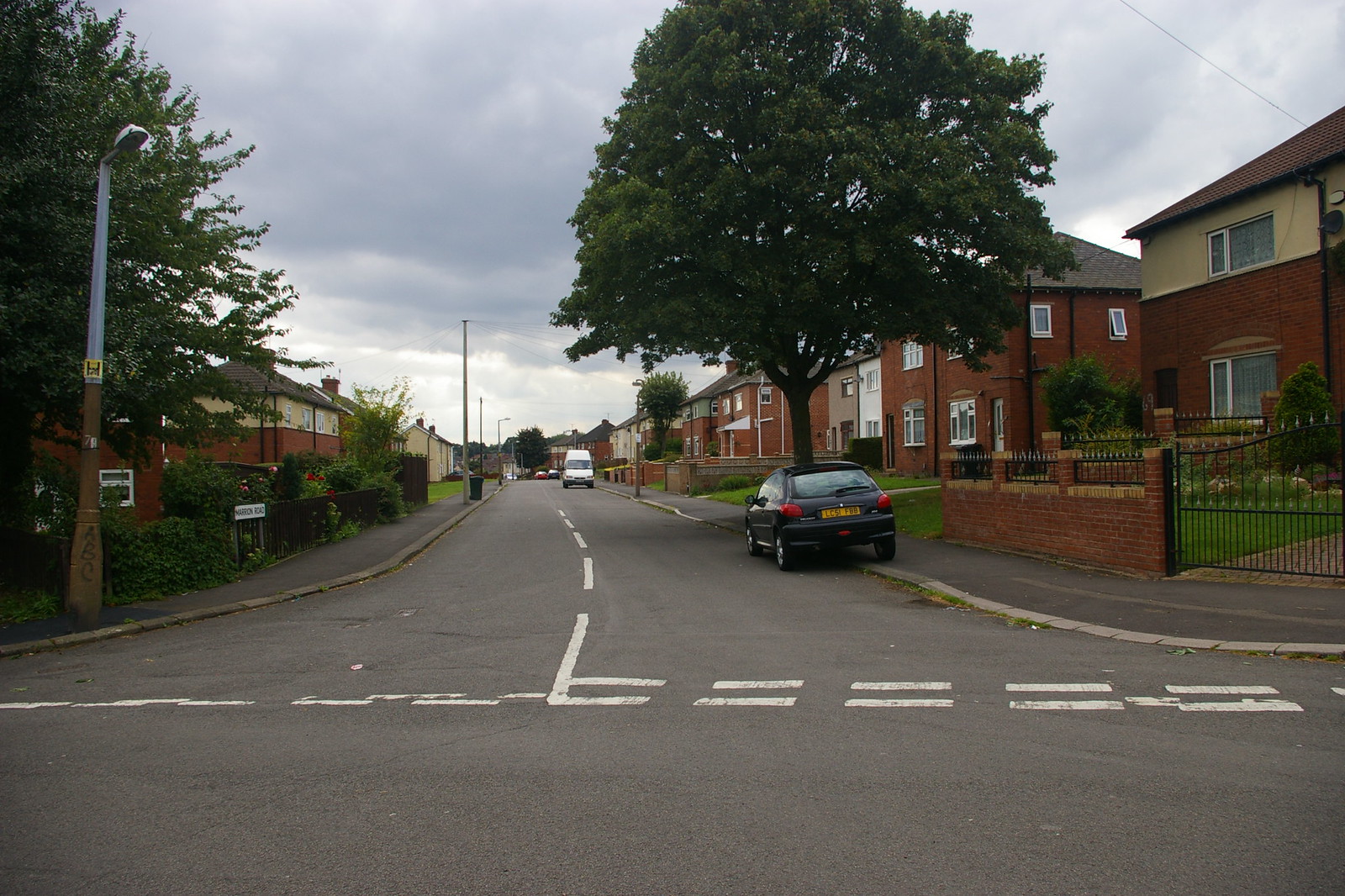The image captures a street scene viewed from a main road entering an apartment complex street. On the right, a series of two-story homes are visible, featuring red brick or tan facades with brown, tiled roofs. Many of these homes have courtyards enclosed by brick fences with wrought iron gates. The first house is brick with a tan top and a brown roof, flanked by a large tree and trimmed with a brick fence and wrought iron gate. Moving further, there are several other brick houses, with one white and tan house among them. 

At the center of the image, a large street tree stands out, its green leaves contrasting with the overcast sky filled with full, grey clouds that suggest impending rain. The street itself is grey with white dashed lines running horizontally and vertically, bordered by sidewalks of varying shades of grey. 

In the foreground on the left side, there's a black trash can and a black gate entwined with green leaves and stems. A streetlamp with a yellow paper attached to it is also prominent. Further down, more houses and streetlights can be seen, with a tan house featuring a wrought iron gate covered in plants and bushes. 

A black car with a yellow license plate is parked half on the street, half on the sidewalk curb. Up ahead, a white delivery van is driving towards the viewer. Overall, the scene is bathed in daylight, with the sun trying to poke through the dense clouds.